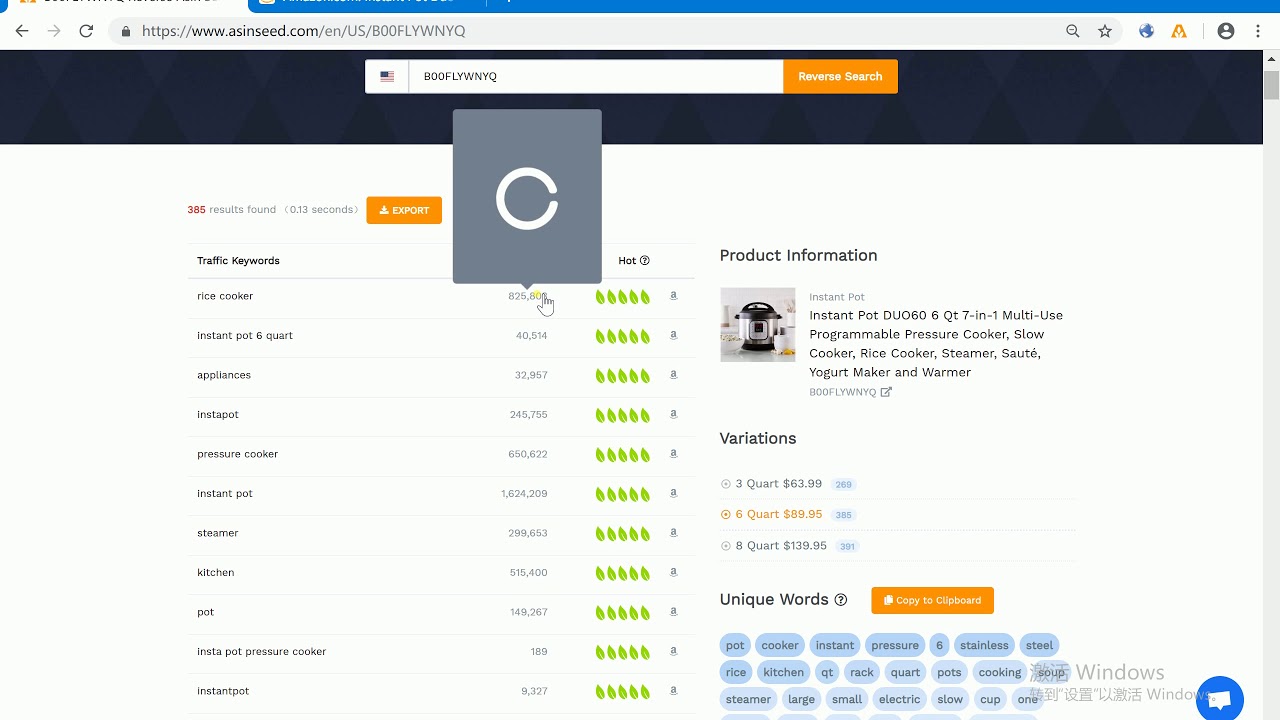The image is a screenshot of a computer screen displaying a search result page from the website www.asinseed.com-las-booflywnyq. At the top of the page, the URL is entered in the browser's search bar. 

To the left of the search bar is an American flag icon, and on the right is an orange rectangular button labeled "Reverse Search." Below the search bar, the URL is also inputted again.

The main content area features several elements: a large gray square with a white circle inside that doesn't completely touch the right center area of the circle. To the left, there is another orange rectangle button labeled "Export." 

To the right, a square displays an image of an Instant Pot, showcasing a silver and black design with a digital screen on its front. Above the Instant Pot image, product information is provided, including the description: "Instant Pot DU060 6-quart 7-in-1 multi-use programmable pressure cooker, slow cooker, rice cooker, steamer, sauté, yogurt maker, and warmer." 

Below the description, variations are mentioned, and another orange rectangular button labeled "Copy to Clipboard" displays the price, listed as "88.80 USD" in orange.

The page also includes a section labeled "Unique Words."